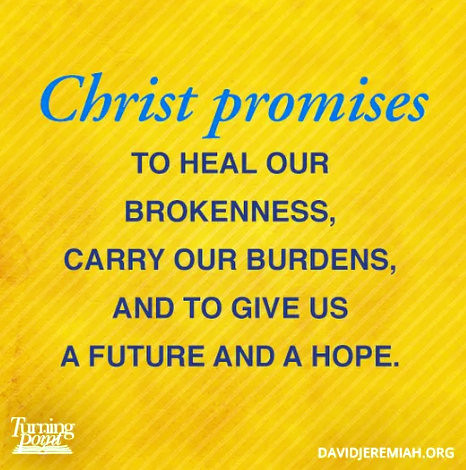The image depicts a small, simple print piece resembling a business card. It features a yellow background with a textured pattern of sideways lines that become more pronounced towards the center. The top of the card showcases the phrase "CHRIST PROMISES" in bright blue capital letters. Following this, in dark blue capital letters, is the message: "TO HEAL OUR BROKENNESS, CARRY OUR BURDENS, AND TO GIVE US A FUTURE AND A HOPE." The lower left corner contains the white logo of Turning Point Ministries, and the lower right corner displays the website "DavidJeremiah.org" in white text.